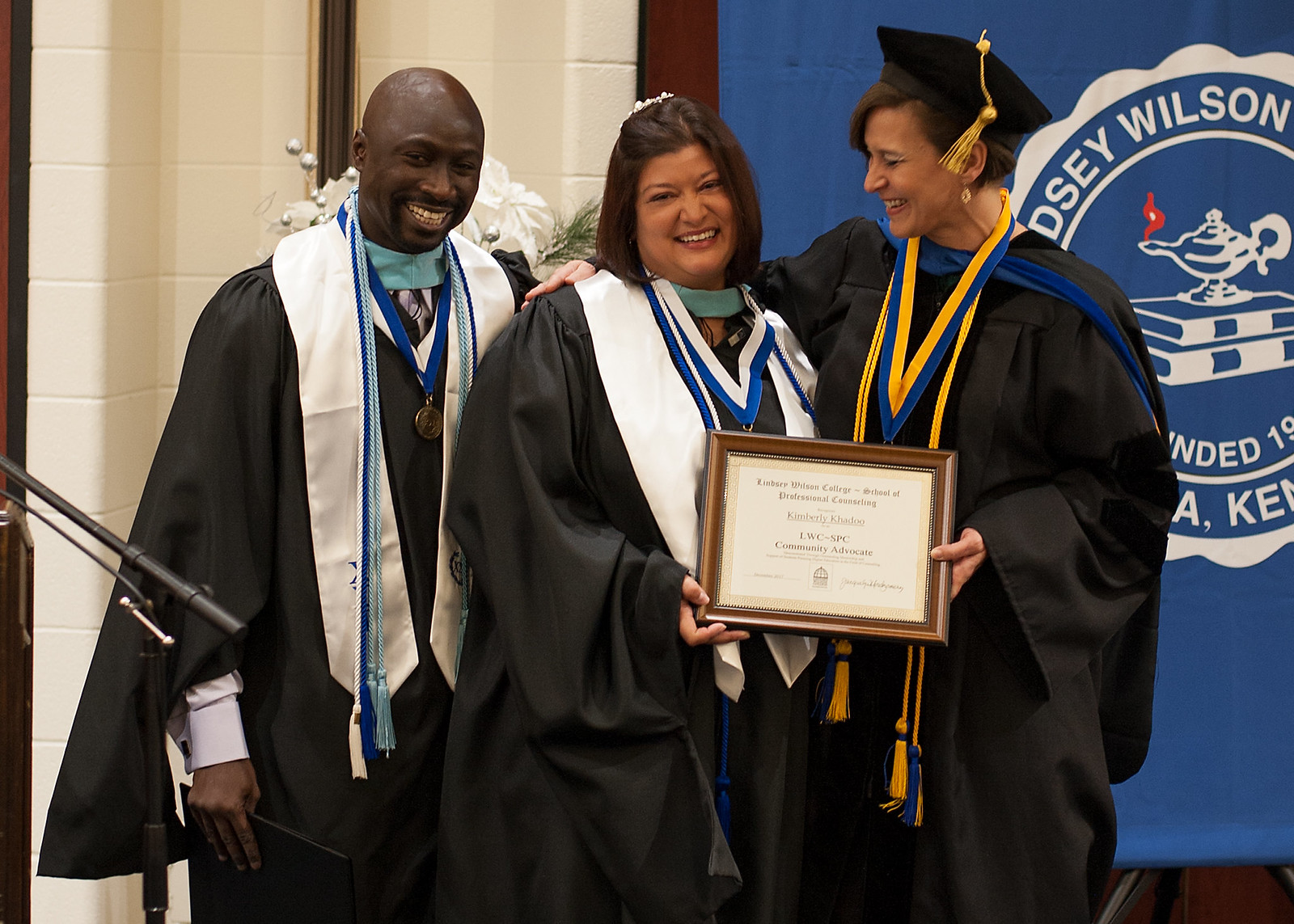The photograph captures a group of three individuals dressed in ceremonial academic robes, seen from the knees up, standing in front of a backdrop featuring a white, stone cinder block wall on the left and a large banner with a circular logo and white text on the right. The leftmost person is a bald man wearing a long-sleeve purple shirt beneath a black robe, accessorized with a white scarf, a blue ribbon with a gold medallion, and he appears to be smiling. Beside him stands a woman with short black hair, donned in a black robe and a white scarf, with a black and white ribbon holding a medal. She holds the corner of a brown framed certificate featuring black text on white paper. The third individual, to her right, is a woman wearing a square academic hat with yellow tassels, also dressed in black robes. She wears a yellow and blue pendant. Both women are holding the framed certificate together. The trio appears to be celebrating a significant academic achievement.